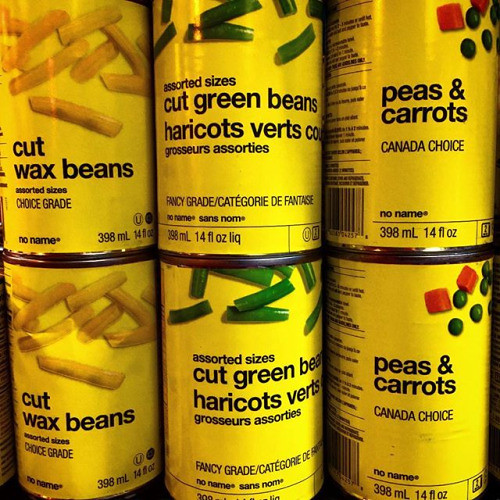The image displays six identical bright yellow cans, arranged in two neat rows. Each can features black lettering. The top three cans from left to right are labeled as follows: The first can says "Cut Wax Beans," "Choice Grade," and shows an image of yellow wax beans. The second can displays "Cut Green Beans," "Fancy Grade," with a picture of assorted sizes of green beans. The third can is marked "Peas and Carrots," "Canada's Choice," accompanied by an image of green peas and red carrot squares. The bottom row mirrors the top row: "Cut Wax Beans," "Cut Green Beans," and "Peas and Carrots" again. Below each product name at the bottom, it states "No Name" to indicate the brand, and the can size is listed as 398 milliliters or 14 fluid ounces. The uniform yellow design and consistent labeling suggest these are budget-friendly, basic canned vegetables.